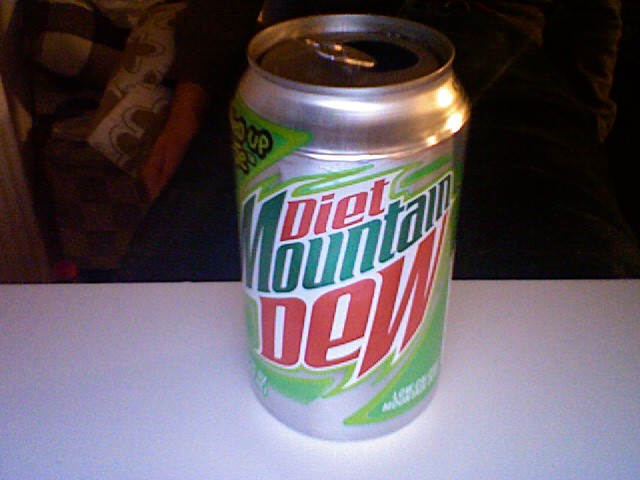This image features a close-up of an open aluminum can of Diet Mountain Dew, prominently positioned in the center of the frame on a plain white counter. The can is decorated with the typical Mountain Dew logo: "diet" in red, "Mountain" in green, and "Dew" in red, all outlined in white with sharp, pointed accents. The design includes a green triangle at the top left of the logo with the partially legible word "up." The pop tab is visibly lifted, revealing a bit of soda on the lip of the opening. In the lower right part of the can, there is text indicating the low-calorie content, although the ounces information is blurred and unreadable. The background is predominantly dark, possibly containing some indistinguishable fabrics or pillows in the upper left corner, adding a sense of depth and contrast to the image.